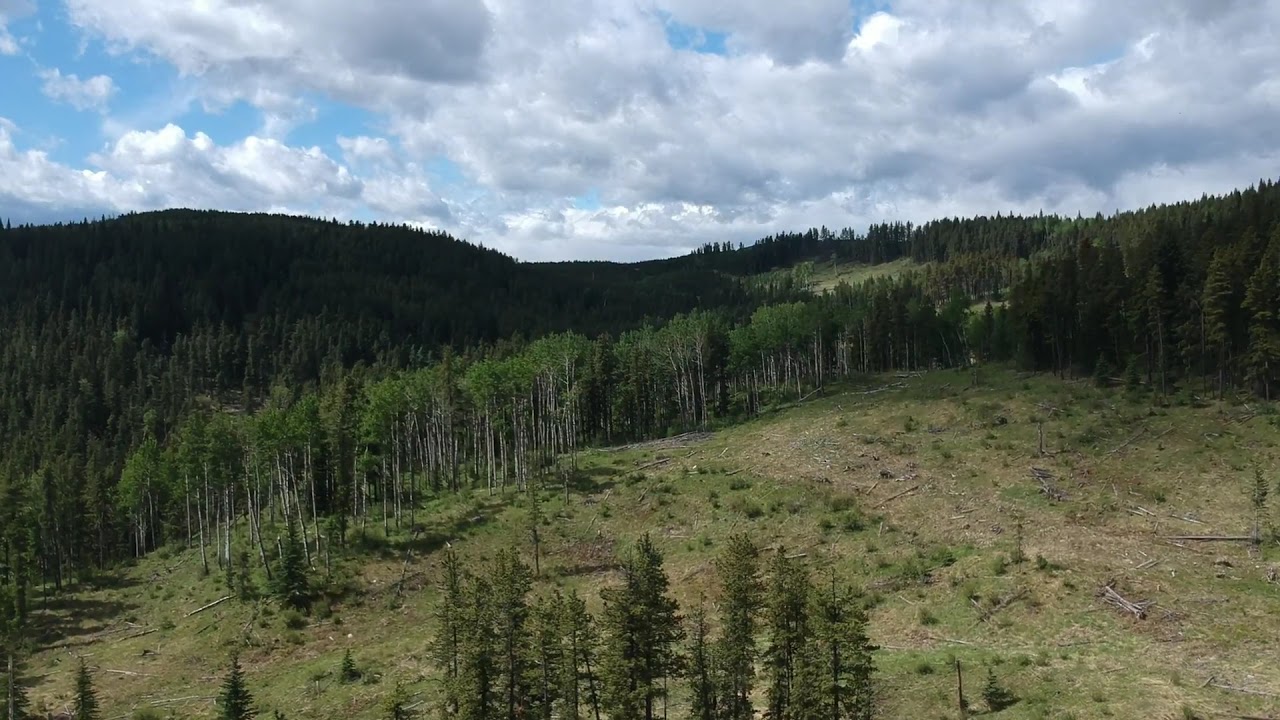This image presents a stunning daytime view of a national forest or park, characterized by a vast and slightly rolling mountainous landscape. In the foreground, we see a grassy and somewhat rocky hill with dead, fallen logs scattered across it, suggesting recent logging activity. The grassy terrain includes patches of green and light tan grass interspersed with tree stumps and logs. On the lower right side, the landscape appears as an almost clear cross-section of forestry work.

As the perspective shifts upward, tall trees with light-colored, almost white trunks rise prominently from the top of the hill. These trees boast foliage mainly concentrated at their tops, creating dramatic, silhouetted outlines against the sky. The hill in the distance is shrouded in shadow, rendering the trees almost black along the skyline.

Dominating the upper half of the picture is a brilliant blue sky adorned with thick, white puffy clouds with darker undersides, adding depth and contrast to the serene scene. The combination of vibrant natural elements and subtle signs of human activity paint a comprehensive picture of this tranquil yet dynamic outdoor habitat.